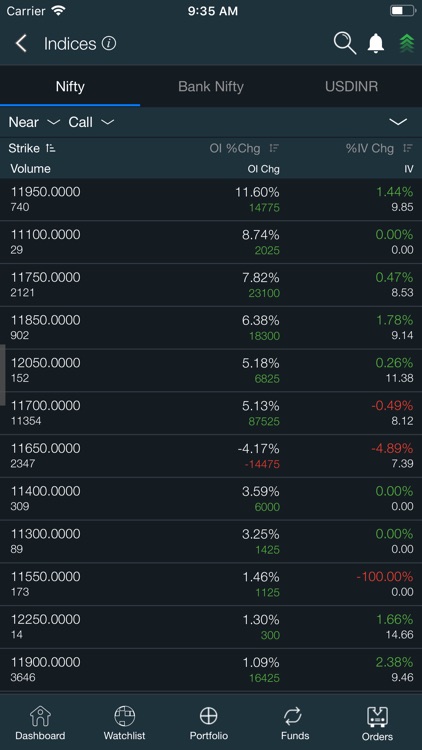Screenshot of a Mobile Stock Portfolio Dashboard:

The image is a mobile phone screenshot displaying a stock portfolio index at 9:35 AM. The phone's battery is at half capacity. In the header, the word "Indices" is shown next to a back button. Below the header is a menu with options: Nifty, Bank Nifty, and USDINR, with Nifty currently selected, indicated by a blue underline. 

The background is black with white text, highlighted with green and red colors to signify increases and decreases in prices, respectively. The page is organized into three main columns:

1. Strike Volume
2. Percent Change (OI Percent Change)
3. IV Percent Change

Several rows of data represent different strike volumes under these columns.

At the bottom of the screen are navigation links to Dashboard, Watchlist, Portfolio, Funds, and Orders.